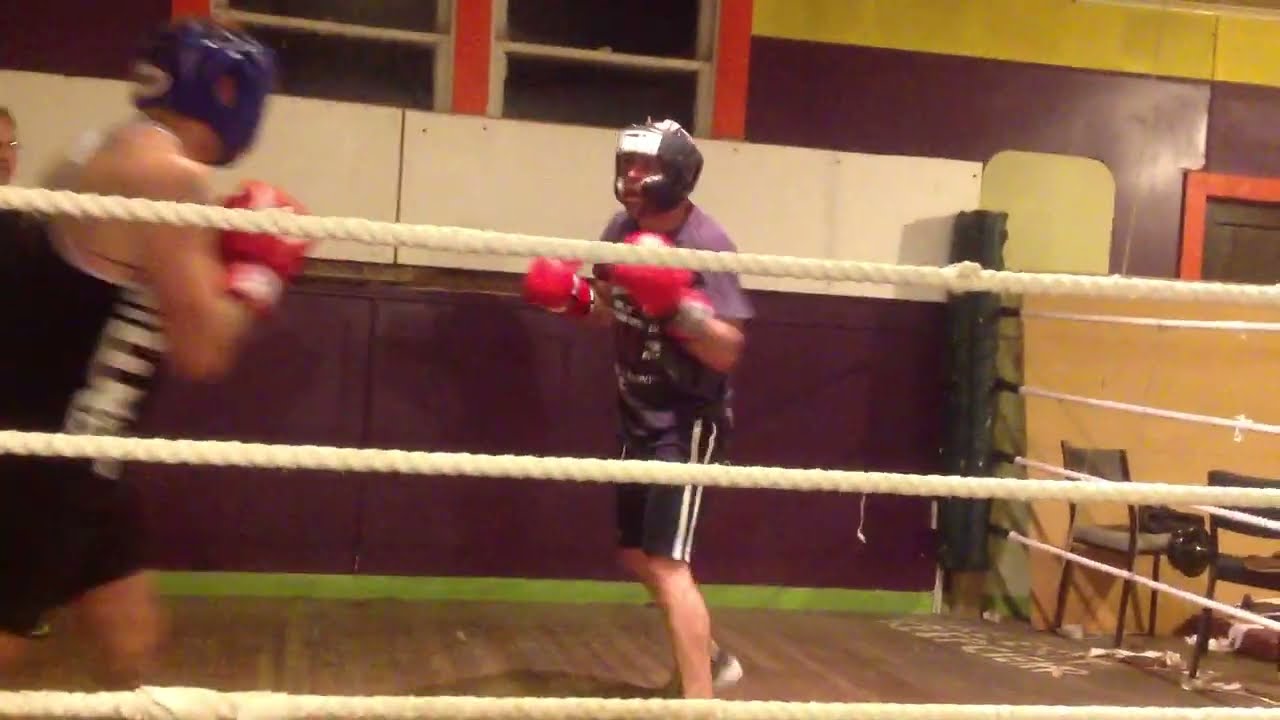This detailed color photograph captures an indoor boxing scene in a small gym. Two boxers are positioned in the ring, partially enclosed by tan ropes visible in the foreground and along the right side, but notably absent behind them. The backdrop features a predominantly purple or eggplant-colored wall with two closed windows, separated by orange vertical stripes. A large white horizontal section, possibly padded, is also part of the background. 

The boxer on the left is equipped with blue headgear, and dressed in a black tank top and black shorts. His opponent on the right sports black headgear, a purple shirt with some obscured lettering, and black shorts with two white vertical stripes. Both fighters are wearing red boxing gloves and are engaged in active sparring, circling one another.

The gym, which appears more like a training facility than a professional arena, has a wooden slat floor. To the right of the ring, two chairs are turned away, adding to the casual, practice atmosphere. The upper left corner of the image just captures the partial face of a man with glasses, possibly a coach or referee, in front of the white padded section of the wall. Overall, the scene highlights a focused training session with a vibrant and slightly worn-in gym setting.